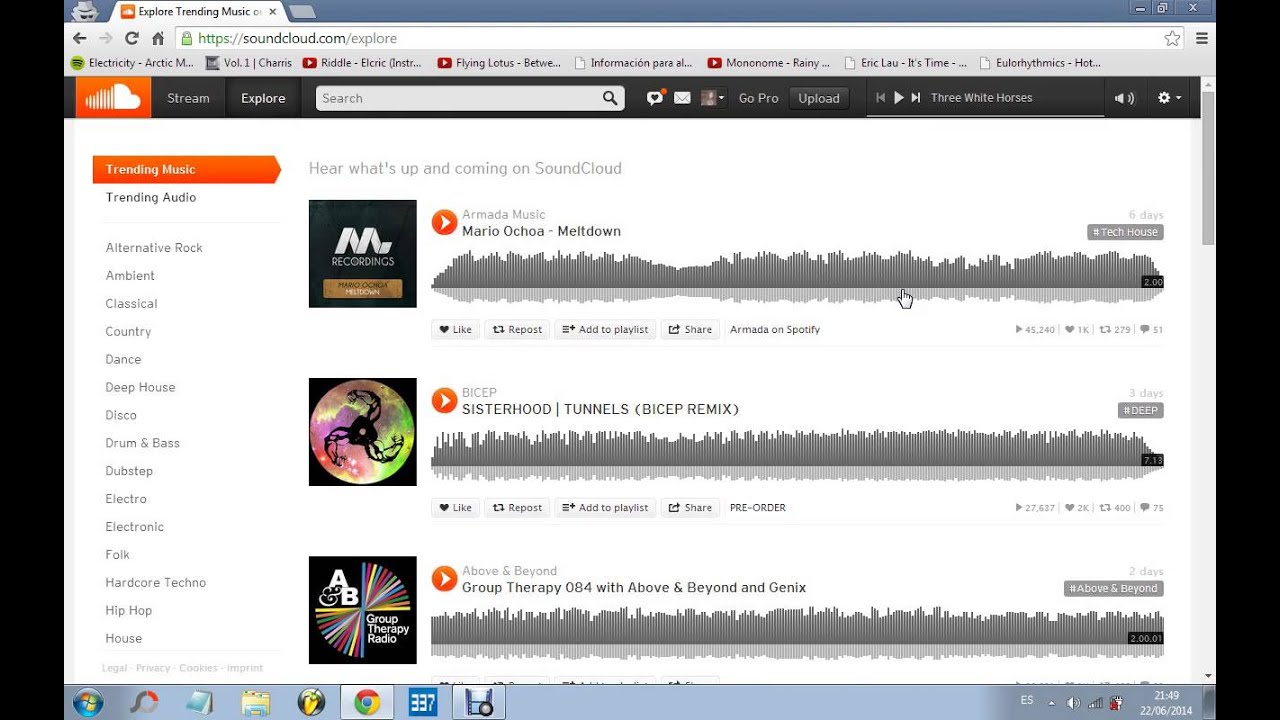Here is a cleaned-up and detailed caption for the described image:

---

This image showcases an incognito web page of the music platform SoundCloud. At the top of the page, the header reads "Explore Trending Music," and the URL in the address bar is "soundcloud.com/explore." Below the header, several trending music tracks are listed, including "Electricity Arctic Volume One," "Chains," "Reddit," and "Flying Lotus." These entries are accompanied by various icons, including YouTube icons, and some information represented by ellipsis marks.

The SoundCloud emblem is visible in the navigation bar along with options to Explore, Stream, and a search bar. To the right of these options are buttons labeled "Go," "Pro," and "Upload." Beneath this navigation bar, the page offers categories of trending music, such as "Trending Music," "Trending Audio," "Alternative Rock," "Ambient," "Classical," "Country," "Dance," "Deep House," "Disco," "Drum & Bass," "Dubstep," "Electro," "Electronic," "Folk," "Hardcore," "Techno," "Hip Hop," and "House." 

The section titled "Here's What's Up and Coming on SoundCloud" features tracks like "Mario Ochoa - Meltdown," "Sisterhood - Tunnels (Bicep Remix)," and "Group Therapy 084 with Above & Beyond and Genix." At the bottom of the page is a toolbar displaying icons for Windows, Notebook, Folder, Google Chrome (version 337), an unspecified application, sound settings, and Wi-Fi or internet connection status. A timestamp at the bottom-right corner reads "21:42, 22-06-2014."

---